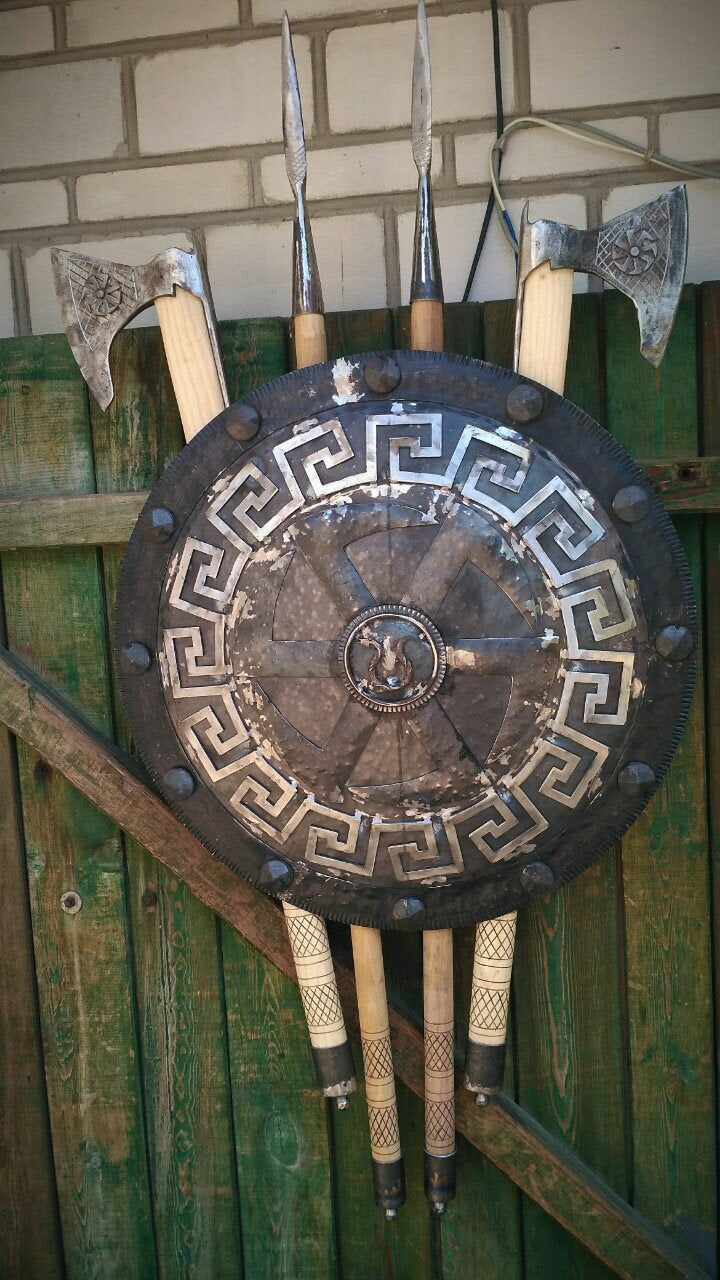The image is a photograph capturing an arrangement of medieval weaponry mounted on a weathered wooden plank door that has been painted green, though the paint is noticeably worn off. The door features a crossbeam running diagonally from the top left to the bottom right. Positioned against the wall of large white bricks, held together with dark gray mortar, the door is slightly ajar, revealing a black and white wire running down from the top center of the image behind it.

The central focus is a large, round black shield adorned with silver studs around its rim and intricate angular patterns forming concentric circles. At its center, there's an emblem reminiscent of an upside-down Omega symbol. Flanking the shield are two axes on the outer edges; each axe has a wooden handle and a metallic head with the blades facing outward—the left axe's blade points left and the right one's blade points right. Between the axes are two spears with darker wooden handles and pointed metallic tips extending upwards.